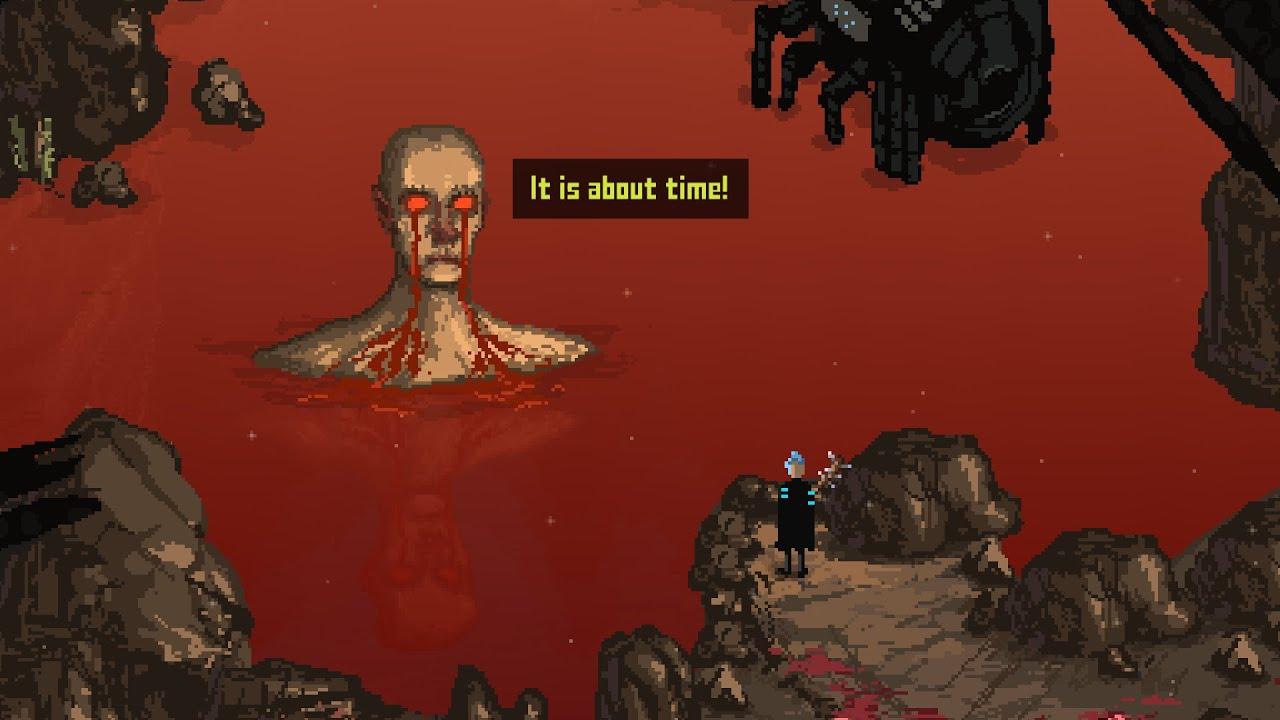In this digital image resembling a 16-bit or 32-bit video game screenshot, a zombie-like creature with blood-red eyes is emerging from a pool of blood that fills the center-left of the scene. The creature's head and shoulders are visible above the crimson liquid, with blood dripping from its eyes. To the right of this menacing figure is a black box with yellow text that ominously declares, "It is about time!" In the upper right corner, a spider-like, robotic creature with sharply angled legs adds to the eerie atmosphere. Meanwhile, on a grey, rocky cliff in the lower right, a smaller character dressed in a black outfit and blue hat stands, gazing directly into the blood pool, seemingly ready for an impending confrontation. Bloodstains scatter across the rocks, heightening the tension as the hero faces the daunting, skeletal adversary.